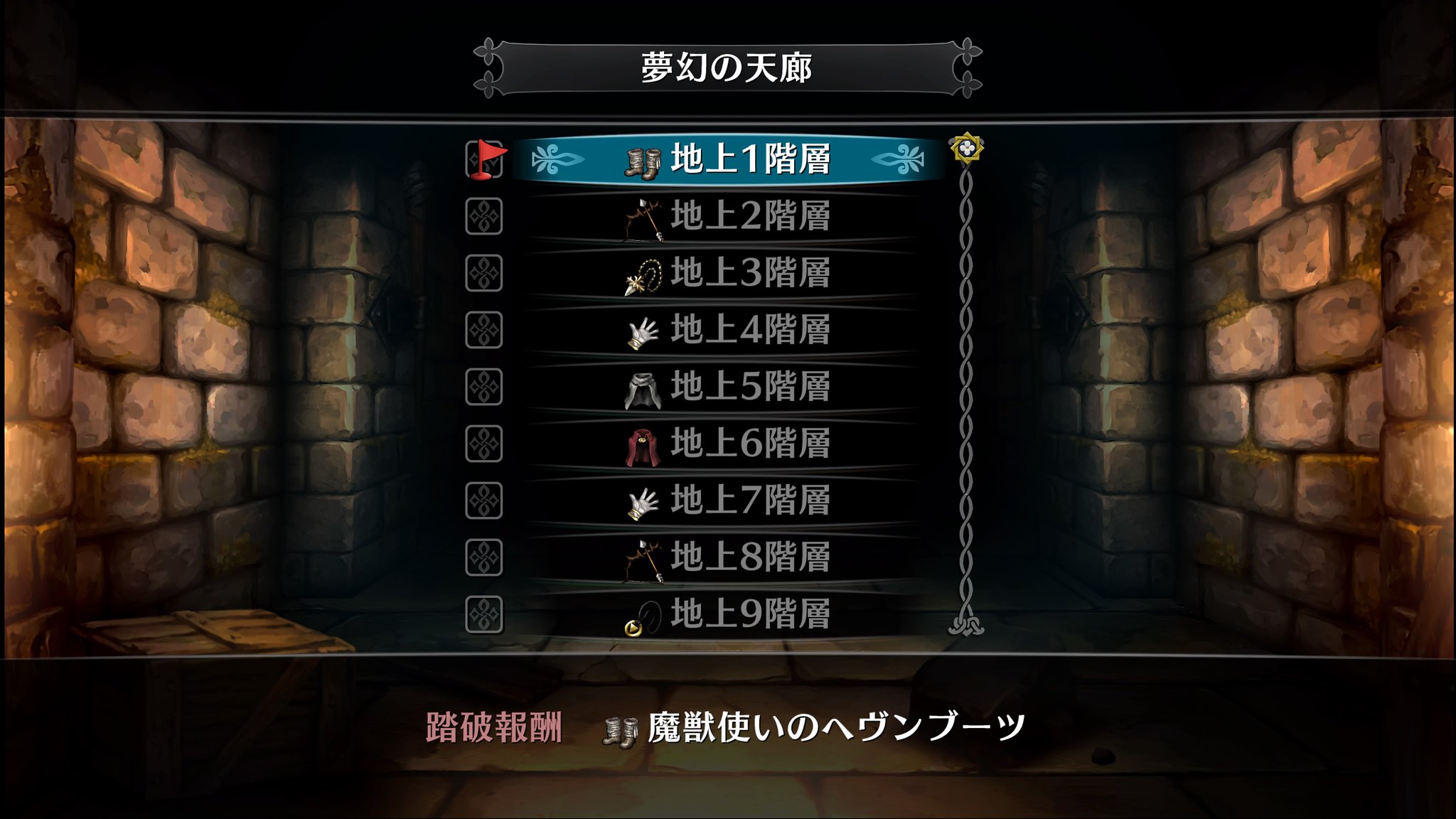This screenshot from a Japanese video game displays a detailed HUD menu situated within a digitally rendered stone room. The walls, in shades of tan, beige, and adorned with patches of green moss, frame the scene on the left, right, and center. At the overall background is predominantly dark with hints of pinkish-gray bricks.

Centrally featured is a menu list filled with Japanese text in white against a black backdrop. The top item in this vertical list is highlighted in cyan blue, contrasting its usual light gray state, adorned with small floral patterns pointing towards it. There is a red flag on the left marking the player's position. On the right, an orange floral spiral is visible above a black rectangle containing more white Japanese text.

The highlighted item in the menu has an icon of a pair of great boots. Following items showcase various game elements: a bow and arrow with silver tips, a gold pendant with a triangular point, a light gray glove with gold cufflinks, a dark gray cape, a maroon cape with a gold centerpiece, another white glove with gold detailing, another bow and arrow, and a circular gold pendant with a black chain. Each item is meticulously depicted, demonstrating the range of available equipment.

At the bottom of the screen, pink Japanese text juxtaposes against the white text above it, indicating additional contextual information about the boots icon at the menu's base. The user interface is punctuated by a highlighted blue top score, enhancing the interactive experience of the in-game environment.